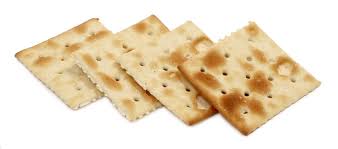This high-quality color photograph features four square crackers, reminiscent of the Jacobs saltine variety typically dunked into soup. Set against a completely whited-out backdrop indicative of professional studio work, the crackers are artfully stacked in a cascading arrangement — the one on the right is perched atop and the stack progressively angles backward to the left. Each cracker displays a grid of air holes, a characteristic feature designed to maintain their flat structure during baking. The crackers are mostly light tan with varying degrees of golden brown patches, particularly pronounced on the topmost cracker, suggesting it spent the most time in the oven. The edges of the crackers feature a subtle, teeth-like design. This close-up shot emphasizes the crackers' crispy and fresh appearance, capturing their slightly different color variations and artful presentation.